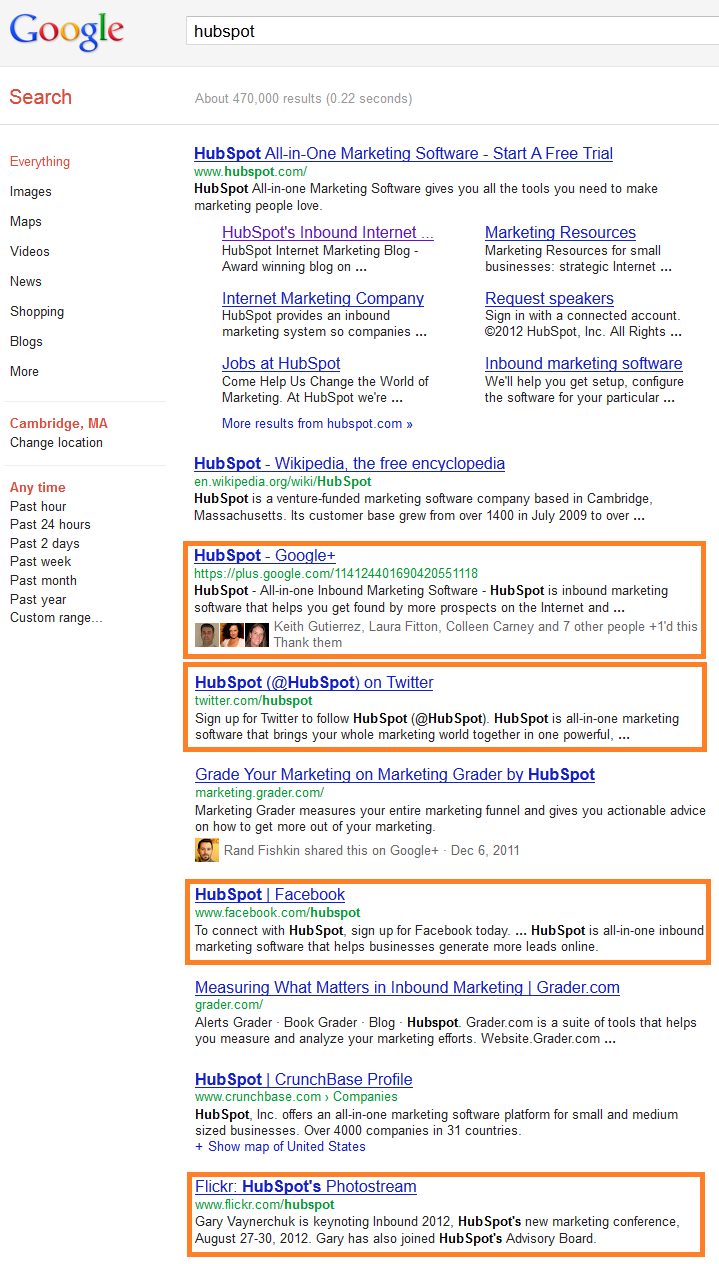The image portrays a Google search results page for the query "HubSpot." In the upper left-hand corner, the Google logo is prominently displayed in its iconic colors: blue, red, yellow, and green. The search bar shows "HubSpot" as the input query. Directly beneath the Google logo, a red "Search" button is visible.

Below the search input are several search filter options highlighted in red, including "Everything," "Images," "Maps," "Videos," "News," "Shopping," "Blogs," and "More." There's an option to change the search location, currently set to "Cambridge, Massachusetts." Additionally, a time filter is available that can be customized to different time frames such as "Any time," "Past hour," "Past 24 hours," "Past week," "Past month," "Past year," and a "Custom range."

The search results show various links related to HubSpot. The first link titled "HubSpot all-in-one marketing software" appears in blue, signaling an unvisited link. Subsequent results include:

- "HubSpot inbound internet marketing resources, internet marketing company, jobs at HubSpot," displayed in purple, indicating previously visited links.
- "HubSpot Wikipedia, the free encyclopedia."
- Boxed links outlined in orange, including "HubSpot Google" and "HubSpot on Twitter."
- A notable snippet that begins, "Read your marketing," mentioning a marketing role at HubSpot.
- "HubSpot Facebook," also outlined in orange, followed by "Measuring what matters in hub and inbound marketing."

Additional references include "HubSpot Crunchbase profile" and "Flickr HubSpot's photostream."

Overall, the image provides a comprehensive look at a Google search results page focused on HubSpot, displaying various resources, social media links, and informational snippets.